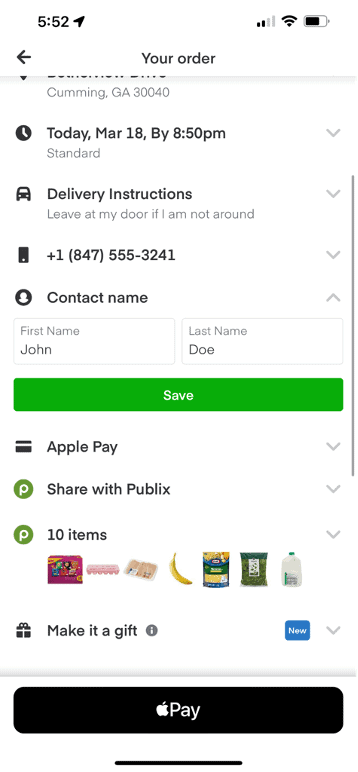A screenshot from a smartphone displayed at 5:52 AM is seen. In the upper left corner, a time stamp reads "5:52," adjacent to which four signal bars appear, with only the first two fully filled. Next to the signal bars are Wi-Fi and battery icons, the latter indicating a half-charged battery. Central to the upper screen, the text "Your Order" is prominently displayed.

Below this header, the screen features a white background indicating delivery tracking. It shows a clock icon accompanied by the text "Today, March 18th, by 8:50 PM," under which "Standard" delivery is mentioned. Below this, a car icon presents specific delivery instructions: "Leave at my door if I am not around." Additionally, a phone icon is linked to the phone number +1-847-555-3241.

Following these details is a contact icon labeled "Contact Name" with two text boxes filled with "John" as the first name and "Doe" as the last name. A prominent green "Save" button is situated below these fields. Subsequently, a dropdown menu indicates "Apple Pay" as the payment method, with the text "Share with Publix" displayed nearby.

Within a green circle to the left is the letter "P," alongside another similar green circle marked "P," indicating the current order includes 10 items. The items listed are visual representations of groceries: chips, eggs, bananas, cheese, and milk. Further down, a gift icon suggests, "Make it a gift."

Finally, at the bottom of the screen, a black Apple Pay button is visible, ready for the user to proceed with the payment.